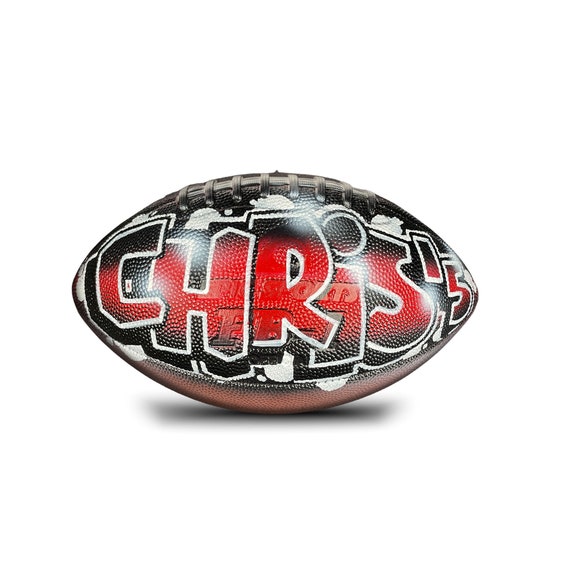The image showcases an American football that has been artistically customized with graffiti-style lettering. The football lies on its side, with the laces positioned upwards and the ends pointing left and right. The primary customization reads "Chris's 5" in bold, red letters with a unique 3D effect created by black and white borders. These letters, which appear as if spray-painted, transition from black at the top through red in the middle to black at the bottom. The background of the football itself is a mix of black and white splotches, with its natural brown leather peeking through at the very bottom. The entire scene is set against a white backdrop, with a subtle shadow beneath the football, adding depth to the image.